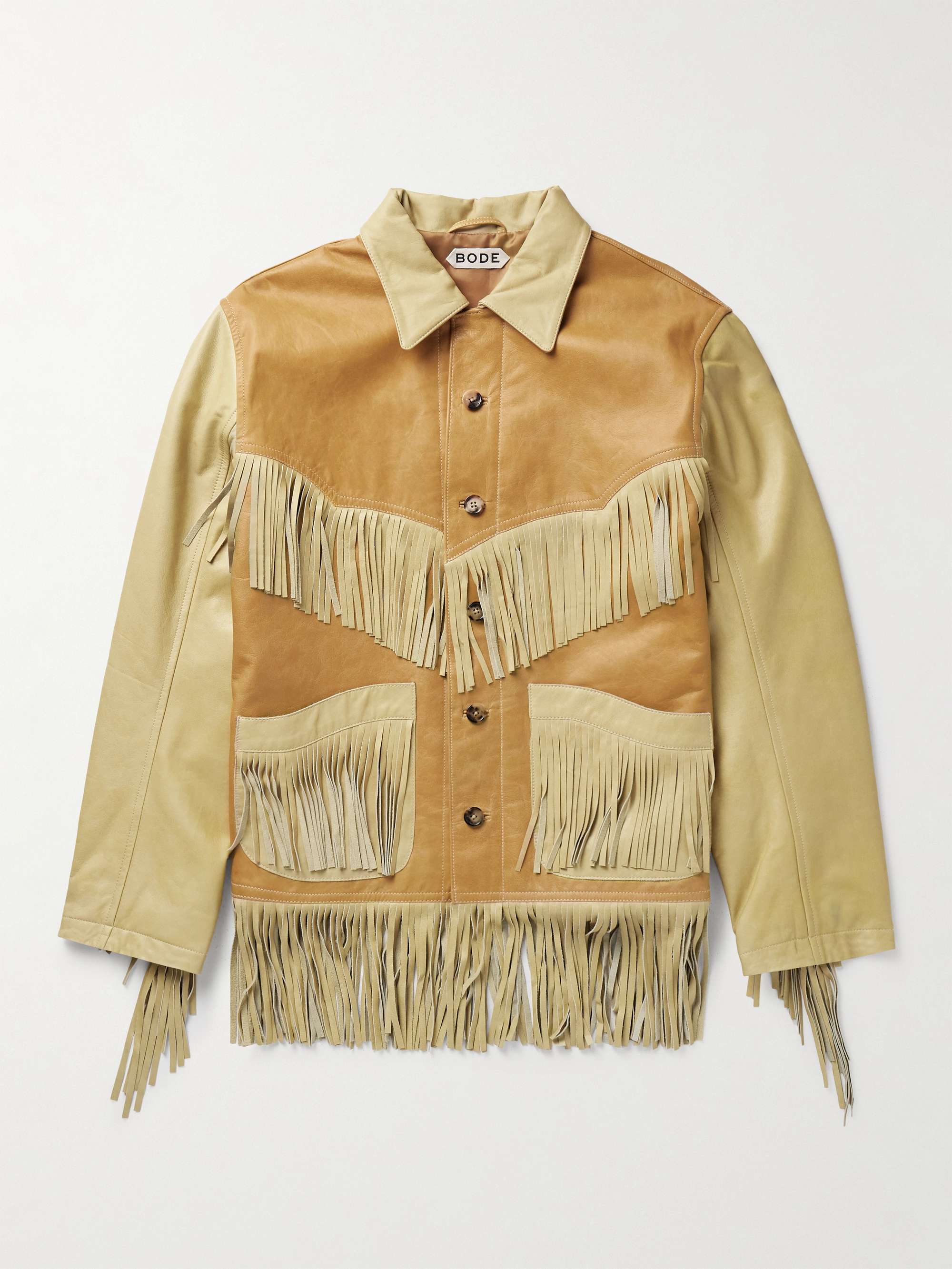The image showcases a distinctive two-tone leather jacket, possibly for women, characterized by a blend of tan and light brown hues. The torso of the jacket is a deeper brown, verging on orange, while the collar, sleeves, and several detailing aspects are in a lighter beige shade. Prominently, the jacket is adorned with fringe or tassel-like strips of leather—which add to its country or desert aesthetic—hanging from the chest pockets, bottom hem, and around the collar, as well as at the ends of the sleeves. It features five tortoise-style buttons that complement its earthy tones. The insider label reads "B.O.D.E" in black lettering on a white tag. The background of the image is white, with the jacket displayed vertically.